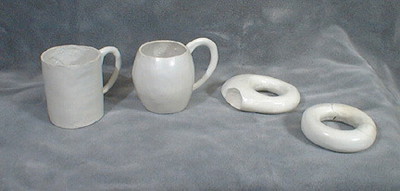This black and white photograph showcases a set of four handmade stoneware pieces displayed on a soft gray cloth, possibly velvet or velveteen. The two white mugs feature distinct shapes: one is thin with straight walls resembling a tin cup, while the other boasts a more rounded, barrel-like form with a narrower opening and a bulbous body. Accompanying the mugs are two circular objects that resemble ceramic donuts; one ring has a distinctive impression or smashed-in section, while the other remains a simple, plain ring. The entire arrangement is rendered in various shades of gray and white, with no additional text or contextual information provided. The photo appears to capture these artisan-crafted pieces in what might be a studio setting.